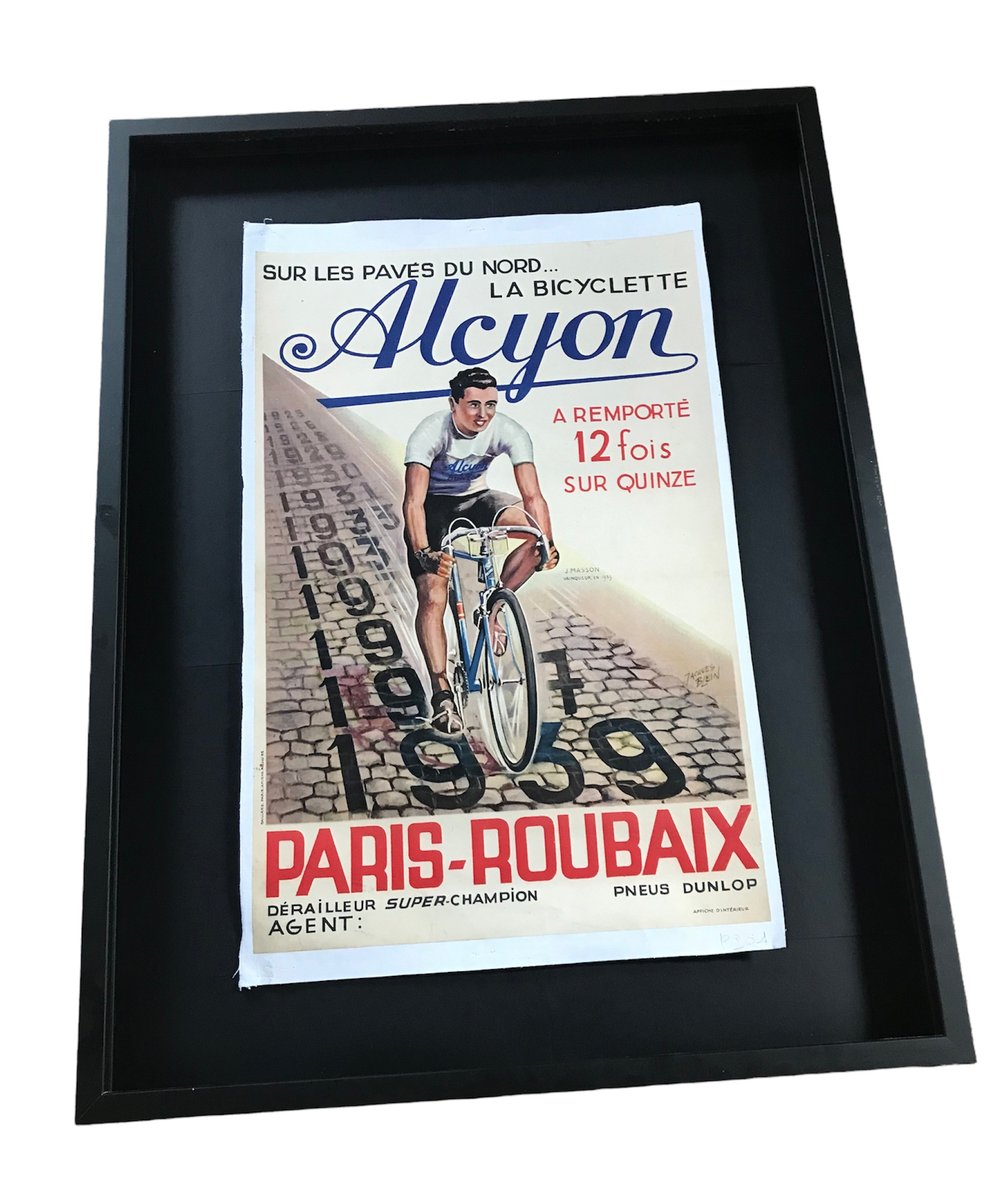This detailed image depicts a framed poster or magazine cover showcasing a classic French cycling theme. The cover, set against a black deep frame, features a predominantly white background intersected by a brick road running vertically down the center. A cyclist, dressed in black shorts, tennis shoes, and a white t-shirt, rides a bike towards the viewer along this road. The road is marked with years like 1939 and 1937, counting down as it recedes.

At the top of the cover, bold black lettering reads "S-U-R-L-E-S-P-A-V-E-S-D-U-N-O-R-D," with "La Biciclette" written just below it. The name "A-L-C-Y-O-N" appears in blue cursive writing underneath these titles. On the right-hand side, red lettering displays "A-R-E-M-P-O-R-T-E, 12 F-O-I-S, S-U-R-Q-U-I-N-Z-E."

Further down, near the cyclist, red lettering spells out "Paris Roubaix," and beneath this, the words "super champion agent" are printed. The overall tone of the poster includes shades of blue, pale yellow, black, red, beige, and gray, all slightly tilted towards the left within the frame. This piece appears to be a promotional or commemorative material for the 1939 Paris-Roubaix Super Champion cycling event.